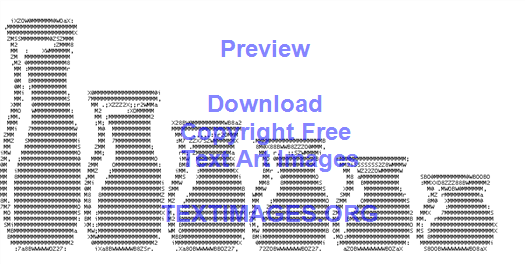The image showcases six vases of varying heights, transitioning from the tallest on the left to the shortest, more rounded one on the right. Each vase appears to be constructed from random characters on a computer, giving them a unique text art style. The vases are filled with a black color, featuring a light shine on their left side. The background is white, enhancing the clarity of the text art. Superimposed over the image is a purple watermark with blue text that reads, "Preview, Download Copyright-Free Text Art Images, textimages.org," indicating this is a sample image from the website. The vases also exhibit a slight blurriness, adding to the artistic effect.